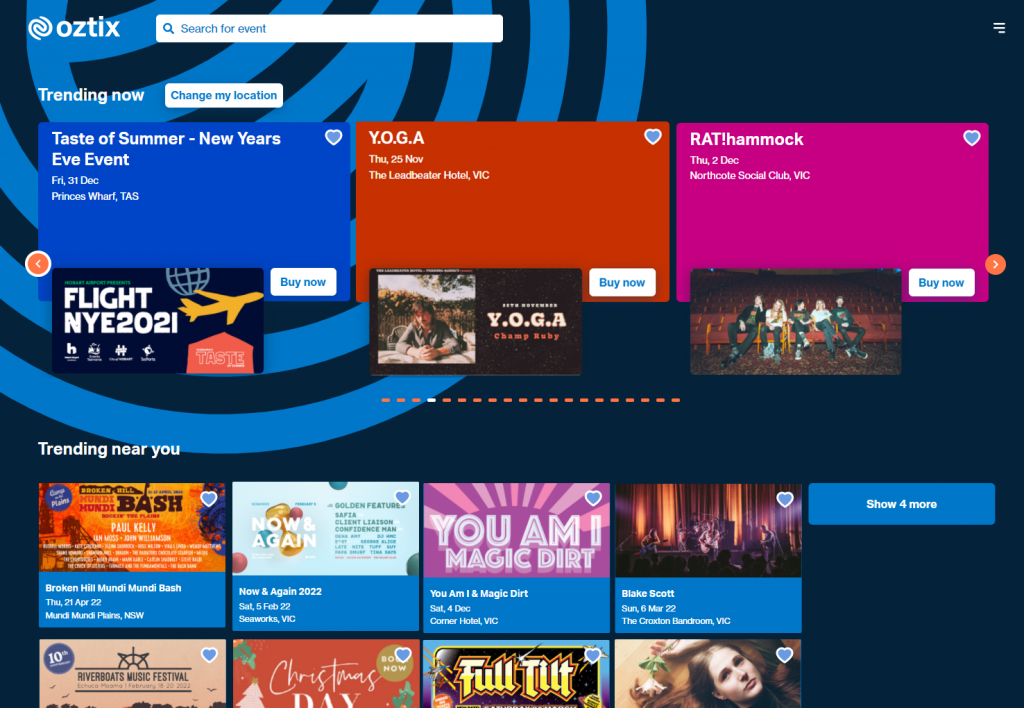The image depicts a webpage for Allstix, showcasing various events. The Allstix logo is positioned at the top left. Below, there is a search bar labeled "Search for event," highlighted in blue. At the bottom of the search bar are options: "Trending Now" and "Change My Location," with the latter also in blue.

Three highlighted events are displayed at the top:

1. **Taste of Summer, New Year's Eve Event**:
   - Date: Friday, 31 December
   - Location: Princess, WAF, TAS
   - Background: Blue
   - Details: Features a "Buy Now" button in blue and white, below which it says "Flight NYE 2021" accompanied by an image of an orange airplane.

2. **Yoga**:
   - Date: Thursday, 25 November
   - Location: Leader Beta Hotel, VIC
   - Background: Red
   - Details: Features a "Buy Now" button at the bottom, with "Save Yoga, Champ Rappi" where "Champ Rappi" is in red.

3. **Red Amok**:
   - Date: Thursday, 2 December
   - Location: North Coast Social Club, VIC
   - Background: Pink
   - Details: Features a "Buy" button and an image of people in a concert hall with red seats.

At the bottom of the main section, under "Trending," events listed include:
- **Broken Hill, Mundi Mundi Bash**
- **Now Again 2022**
- **UMI and Magic Death**
- **Blake Scott**

On the right-hand side, a blue "Show More" button is visible. The overall webpage background is dark purple with a section of blue on the top left.